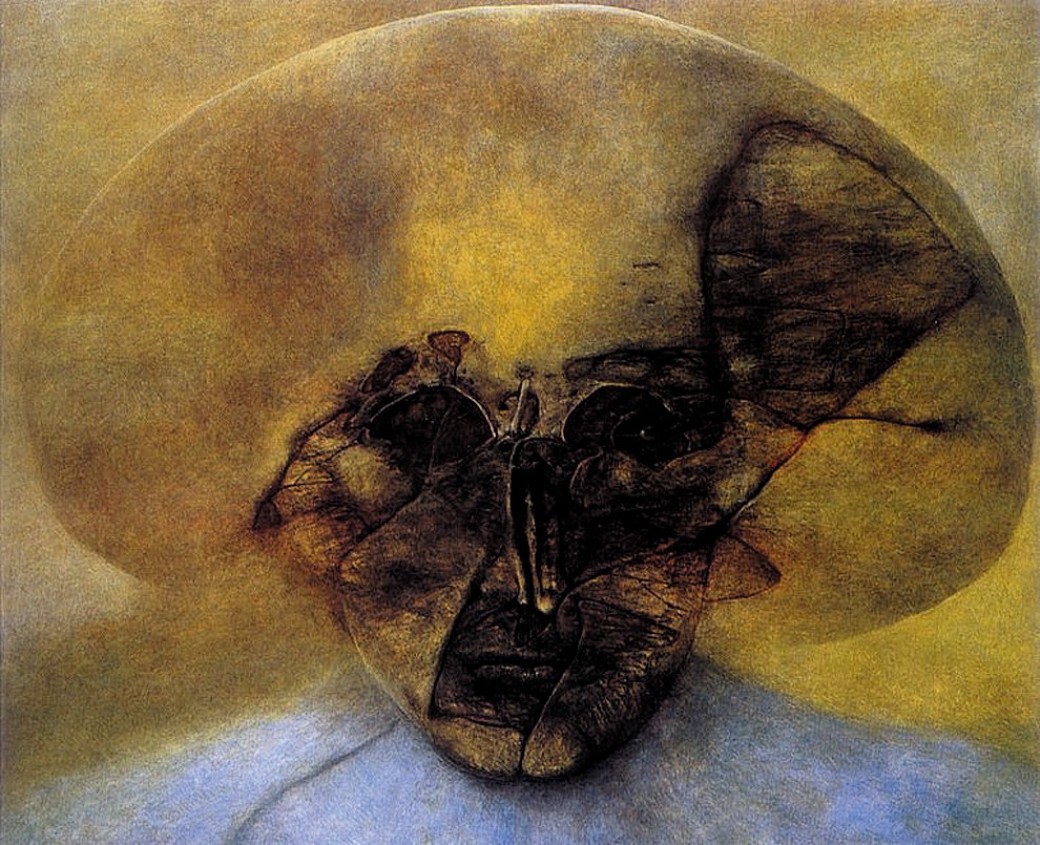The image showcases a highly abstract and surreal painting dominated by hues of yellow, brown, and black, with subtle touches of gray and blue. Central to the composition is a distorted visage resembling a space alien with a mushroom-shaped head, occupying almost the entire canvas. The head, characterized by its mixture of gold, brown, and gray tones, features fractured facial elements that reveal human features beneath. Visible through the cracks are a set of lips and one eye, while the other eye socket appears dark and empty, suggesting a cavity. The nose area is represented by a shadowy void. Over the eyes and nose, there are patterns resembling a bat. The head is portrayed against a background of mustardy yellows and browns, resting on what seem to be abstract impressions of white or gray shoulders. The image emanates an unsettling, almost eerie aura, blending modernist and surrealist styles to create a mesmerizingly peculiar figure.